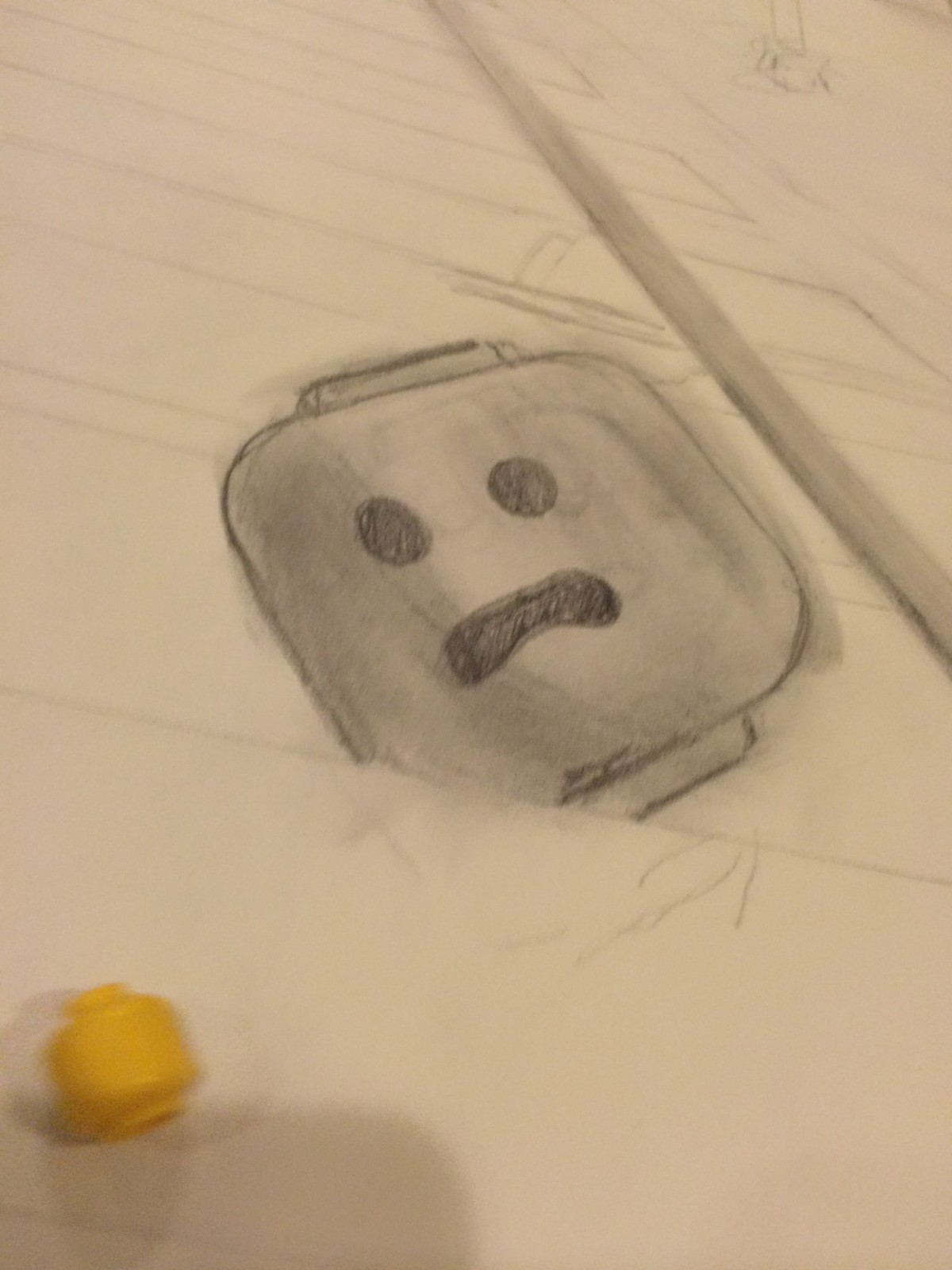The image depicts a detailed pencil sketch in the center of a page, illuminated under tungsten or artificial lighting, giving it a yellowish tint. The drawing features a Lego-like head with a square shape and rounded edges. The head's bottom-left section appears to be erased, giving it an unfinished look. The head has two black, filled-in eyes and an open frown, conveying a sad or scared expression. There is a yellow plastic cylindrical Lego piece positioned at the bottom left corner of the picture, casting shadows. The background of the sketch includes various lines, resembling branches or a grid, adding complexity to the composition and creating an impression of an incomplete and intricate piece of art.